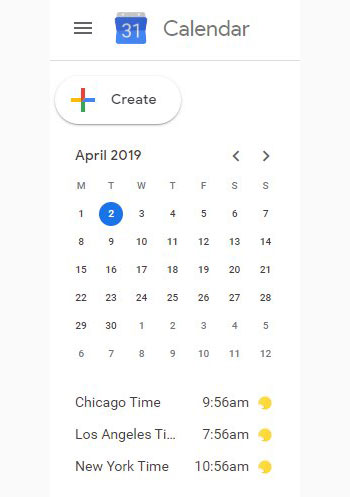The image features a detailed view of a digital calendar interface. At the top left, three horizontal gray lines are visible, followed by a prominent blue calendar icon displaying the number "31" in white. Adjacent to the icon, the word "Calendar" is written in gray. Below this header is a white bar with gray edges, containing a subtle gray line, and a white oval button outlined in gray that reads "Create."

The date shown is April 2019, displayed prominently below this toolbar. To the right of the date, there are left and right arrow icons in gray to navigate through the months. The days of the week are listed in abbreviated form as MTWTFSS. 

Each day of the month is marked within a grid, starting from the 1st at the top and going down to the 12th at the bottom. The 2nd of April is highlighted with a blue circle and a white numeral "2." 

At the very bottom, the calendar shows different time zones: "Chicago time" is at 9:56 a.m., "Los Angeles time" at 7:56 a.m., and "New York time" at 10:56 a.m. Each time entry is accompanied by a half-circle, which appears to be yellow.

Overall, the image provides a comprehensive view of a digital calendar interface, along with specific details, time zones, and navigation elements.